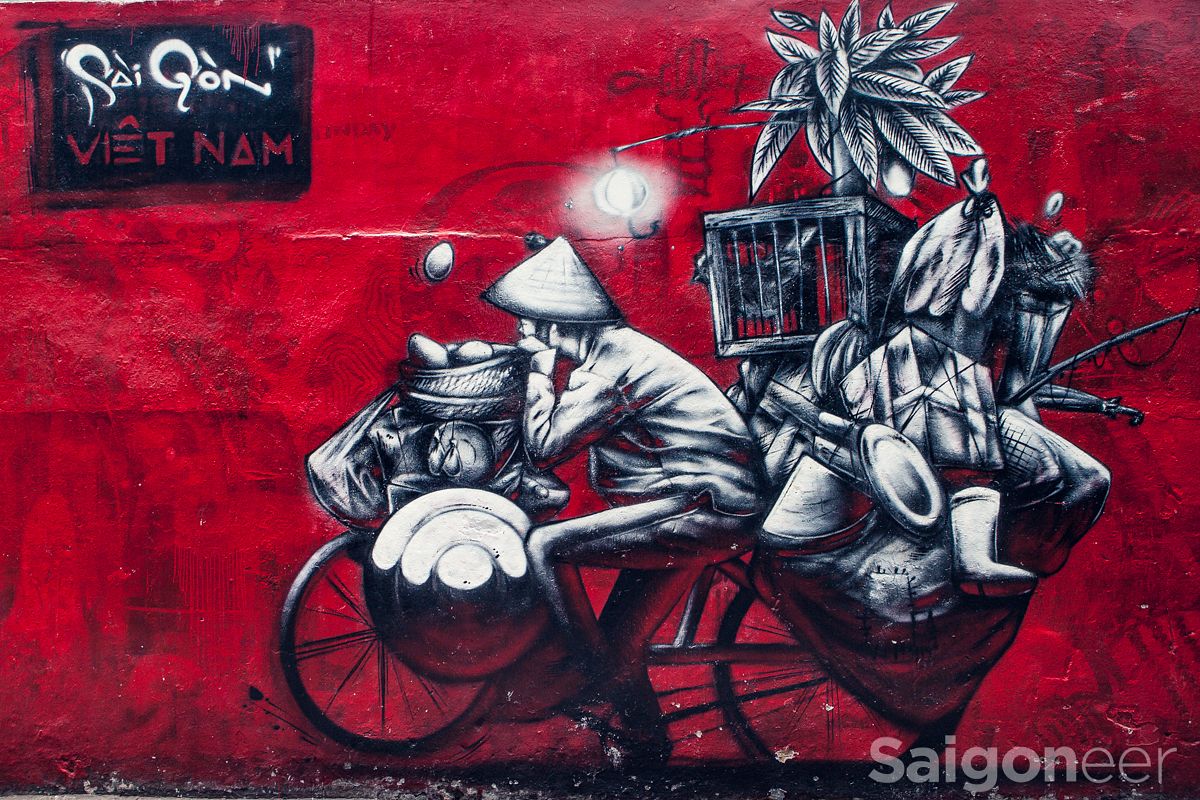This image is a vibrant Vietnamese painting with a striking red background and faint black graffiti-style elements. Dominating the scene, a man rides a heavily laden bicycle. In the top left corner, a black box with white brushstroke text announces "Saigon," with "Vietnam" beneath it in red letters. The man, wearing a pointed hat and possibly a jogging suit, appears either stopped or slowly pedaling. His bike is a marvel of overloading: the front basket cradles eggs, a hubcap, and plastic bags, while the back is an intricate tangle of everyday items. A wooden cage holding a chicken is adorned with flowers, and alongside it are clothes, a plant, a fishing rod, another hat, a plate, a boot, a present box, and various items packed in a bag. The bottom left corner of the painting features the word "Saigonier" in white font, adding a finishing touch to this detailed snapshot of bustling street life in Saigon, Vietnam.